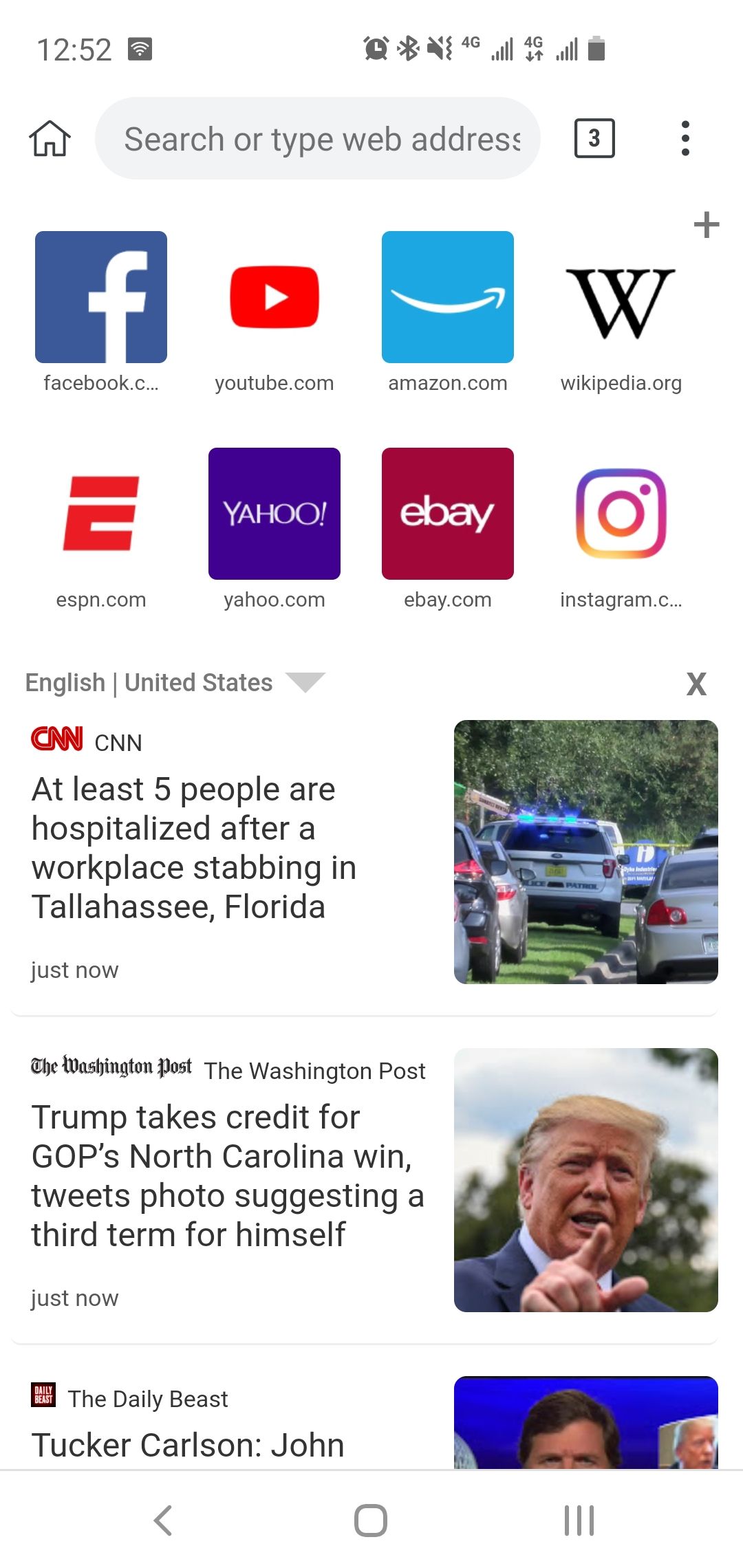A screenshot taken from a smartphone at 12:52 PM displays the browser interface. At the top, there's a home icon followed by a search bar with the placeholder text "Search or type web address." Below the search bar, a row of website shortcuts is visible, each featuring the site's logo above its name: Facebook, YouTube, Amazon, Wikipedia, ESPN, Yahoo, eBay, and Instagram.

Beneath these shortcuts, the screen shows the language setting as "English (United States)" and an 'X' mark at the upper right corner. The bottom section features two news articles. The first, from CNN, has the red CNN logo and reports "At least five people hospitalized after a workplace stabbing in Tallahassee, Florida" alongside an image of emergency vehicles. The second article, from The Washington Post, indicates "Trump takes credit for GOP North Carolina win."